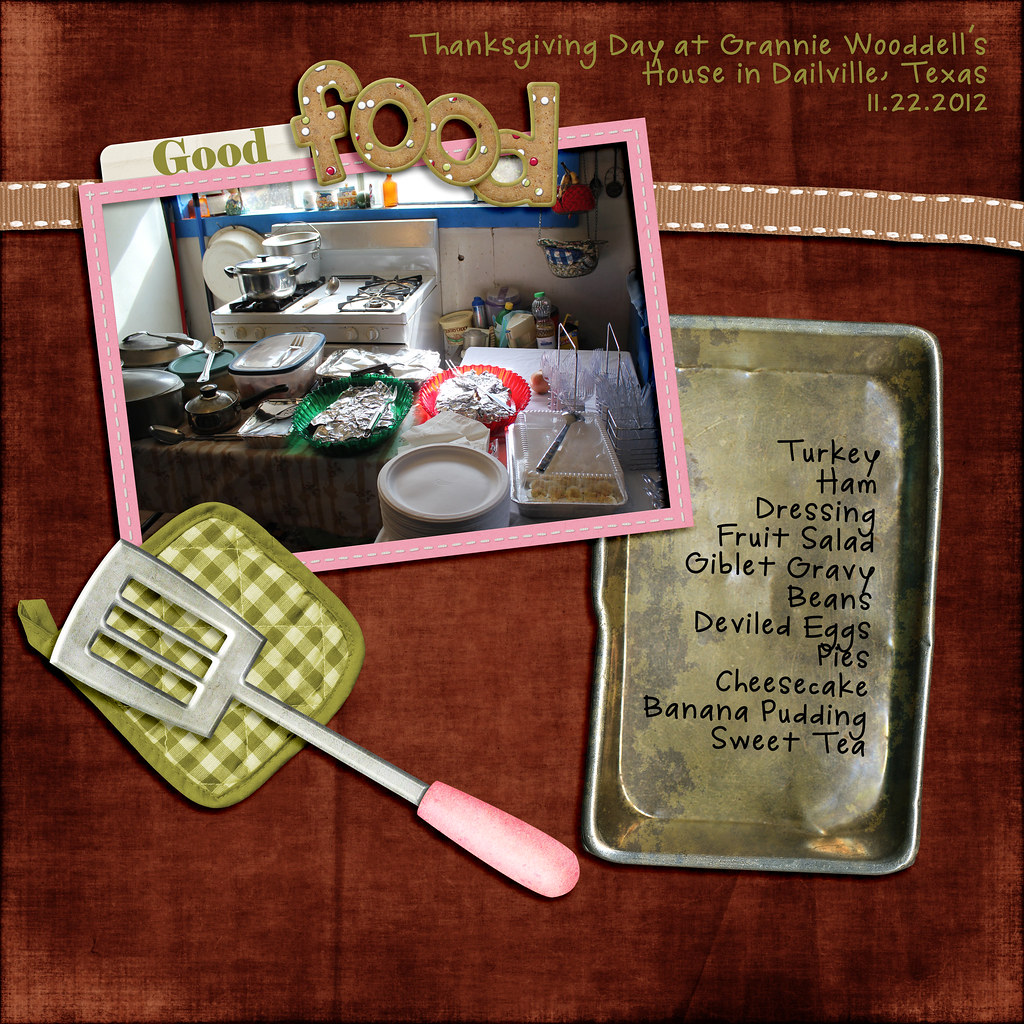The image is a digital scrapbook-styled advertisement for a Thanksgiving dinner, with a rich brownish-reddish background resembling a stained wood table. At the top right, in green and brownish text, it reads "Thanksgiving Day at Granny Wodell's House in Daleville, Texas, 11-22-2012." The centerpiece is a photograph of a kitchen filled with various trays and plates of food, evoking a potluck atmosphere. The photograph is bordered by a pink frame with white dashed lines. Above the photo, it says "good food," with the letters designed to look like fabric scraps, adding to the scrapbook aesthetic. A brown and white dashed ribbon stretches across the image. At the bottom sits a pink-handled metal spatula on a green and white checkered potholder. On the right side, an old metal serving pan lists the menu items in black text: turkey, ham, dressing, fruit salad, giblet gravy, beans, deviled eggs, pies, cheesecake, banana pudding, and sweet tea. The layout and elements convey a nostalgic feel, perfect for sharing on social media.